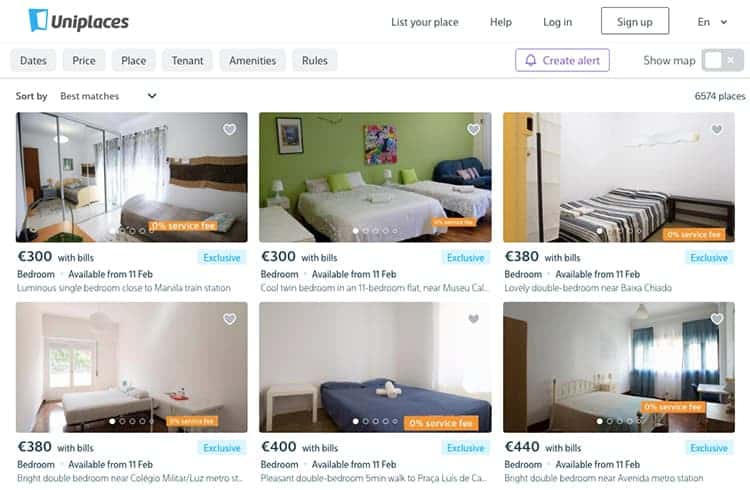The image is a screenshot of a website called UniPlaces, which facilitates room rentals. The website interface allows users to sort listings by various criteria such as dates, price, location, tenant type, available amenities, and house rules. The header menu features options like "List your place," "Help," "Log in," "Sign up," language selection, "Create alert," and "Show map." The displayed listings show six tidy bedrooms available for rent, each furnished with a neatly made bed and appearing like guest rooms. The pricing for the rooms starts at 300 Euros per month, inclusive of certain bills, while one room is listed at 380 Euros per month. The descriptions suggest that bills may include utilities such as electricity and possibly additional services like Wi-Fi. UniPlaces offers a platform for individuals seeking a room in shared accommodations, showcasing options where renters can find a room in someone’s house.